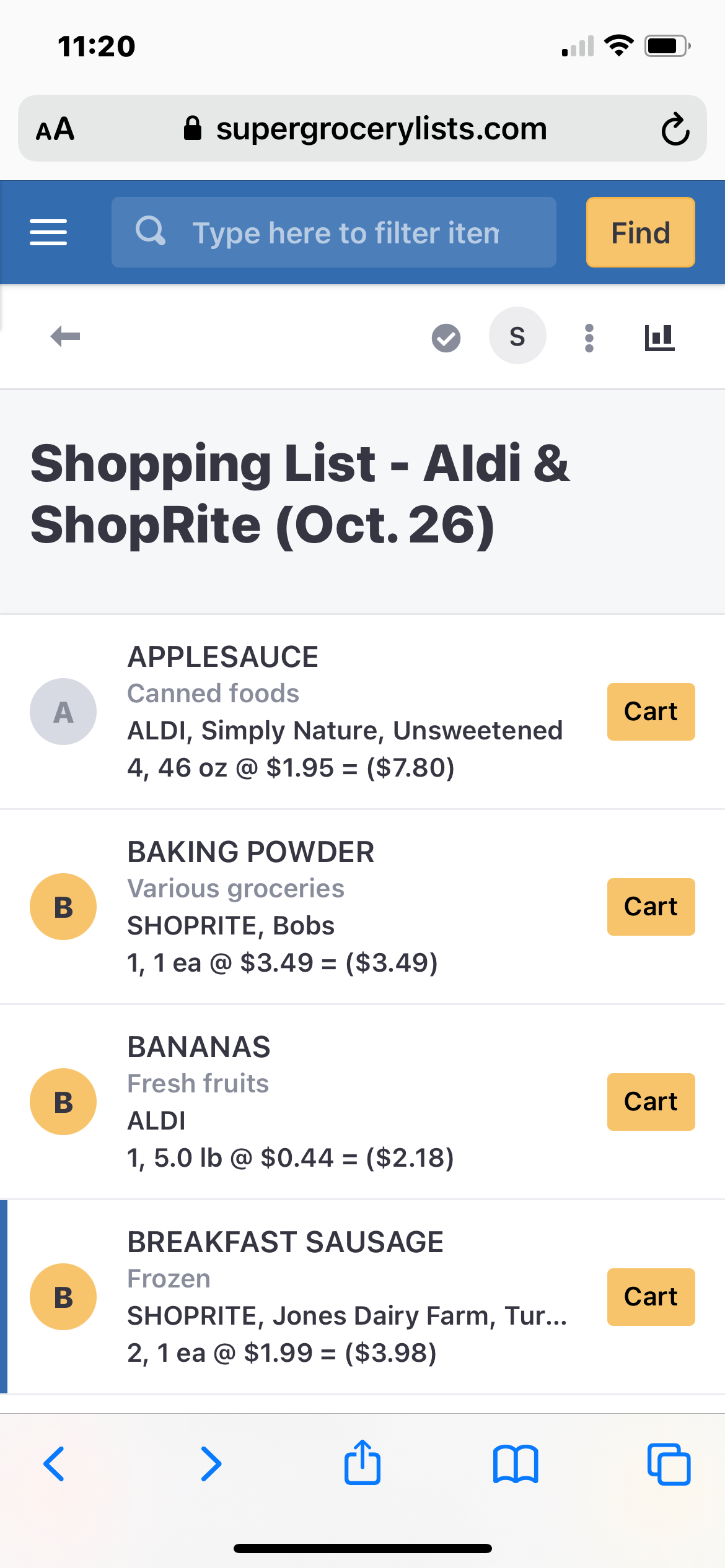The image is a screen grab from a smartphone indicating the time as 11:20 AM with one bar of signal strength and nearly a full battery. The phone's screen displays the website supergrocerylists.com, where the user is organizing their shopping list. The list is titled "Shopping List - Aldi and ShopRite, October 26." 

Detailed items listed are:

1. **Applesauce (Canned)** from Aldi:  Four 46-ounce cans totaling $7.80.
2. **Baking Powder** from ShopRite: One unit priced at $3.49.
3. **Bananas** from Aldi: Five pounds at $0.44 per pound, amounting to $2.18.
4. **Jones Dairy Farm Breakfast Sausage** from ShopRite: Two units at $1.99 each, totaling $3.98.